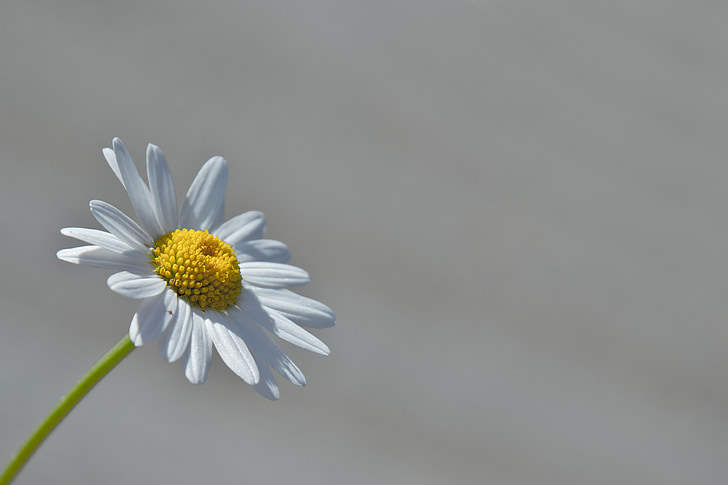This image features a close-up of a single daisy-like flower, distinguished by its green stem and delicate white petals arranged around a vibrant yellow center, densely packed with tiny florets. Emerging from the bottom left corner, the stem curves gracefully upward to about the middle height of the frame, with the flower itself positioned along one of the third lines on the left. The petals reveal intricate lines and indentations, enhanced by the bright light, possibly indicating sunlight, suggesting that the flower might be facing the sun. The background is a plain grayish hue, featuring subtle variations and streaks of darker gray, and the overall lighting hints that this might be an outdoor scene with overcast skies or taken near a window. The composition’s simplicity accentuates the delicate beauty and fine details of the flower, highlighting its potential role as a landing spot for pollinators.